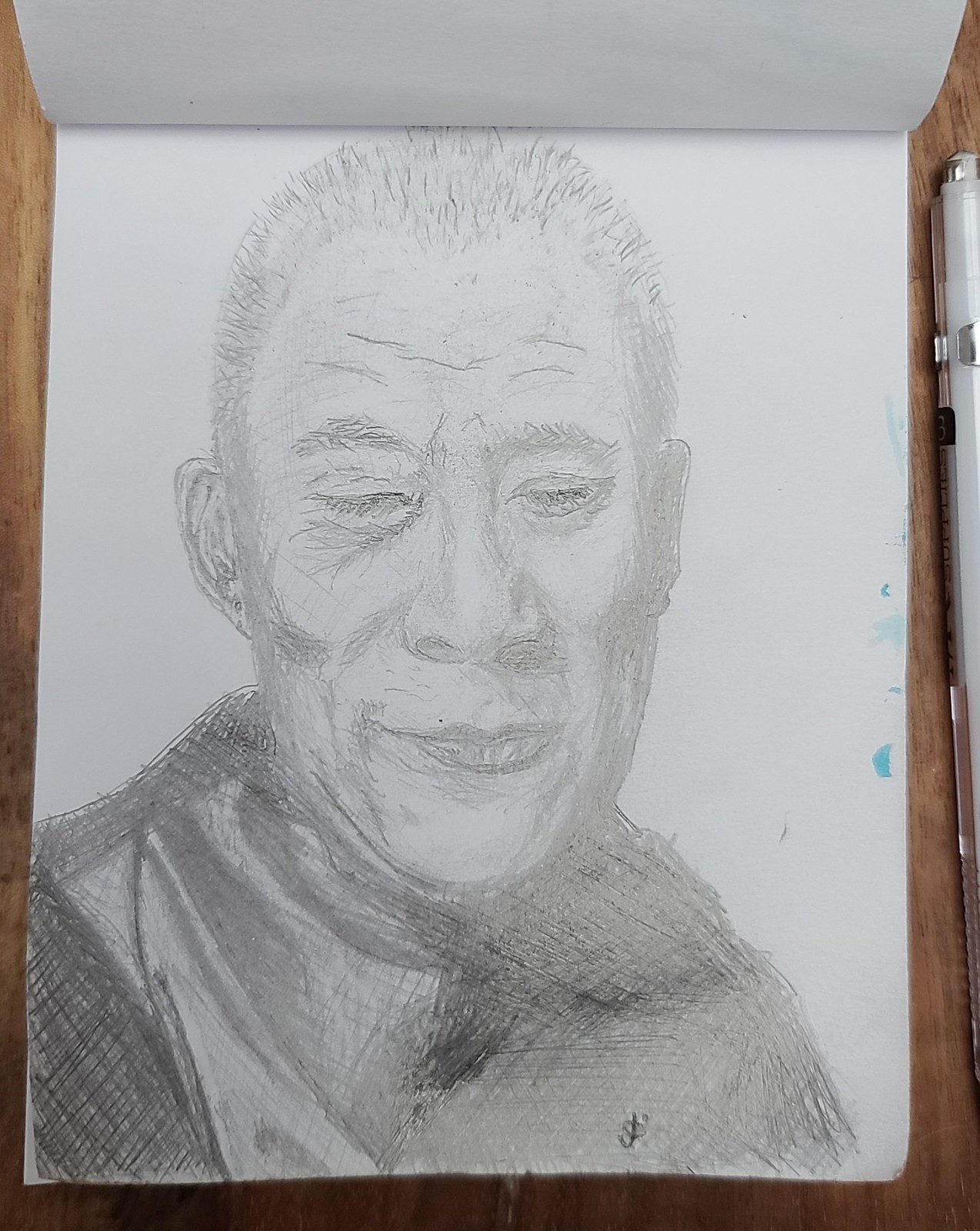This detailed pencil drawing, displayed vertically, features an older man with a serene expression, possibly a famous or religious figure. The man has short, stubbly hair and numerous wrinkles, especially notable on his forehead where five or six lines are visible. His closed eyes and calm demeanor suggest a contemplative state. The drawing, which depicts the man from the shoulders up, shows him with large, flat ears and detailed facial lines, emphasizing his age. The man’s attire, heavily shaded in dark pencil, contrasts with a lighter strip near his left shoulder. The paper, securely placed on a wooden table, shows a slight fold at the top right corner.